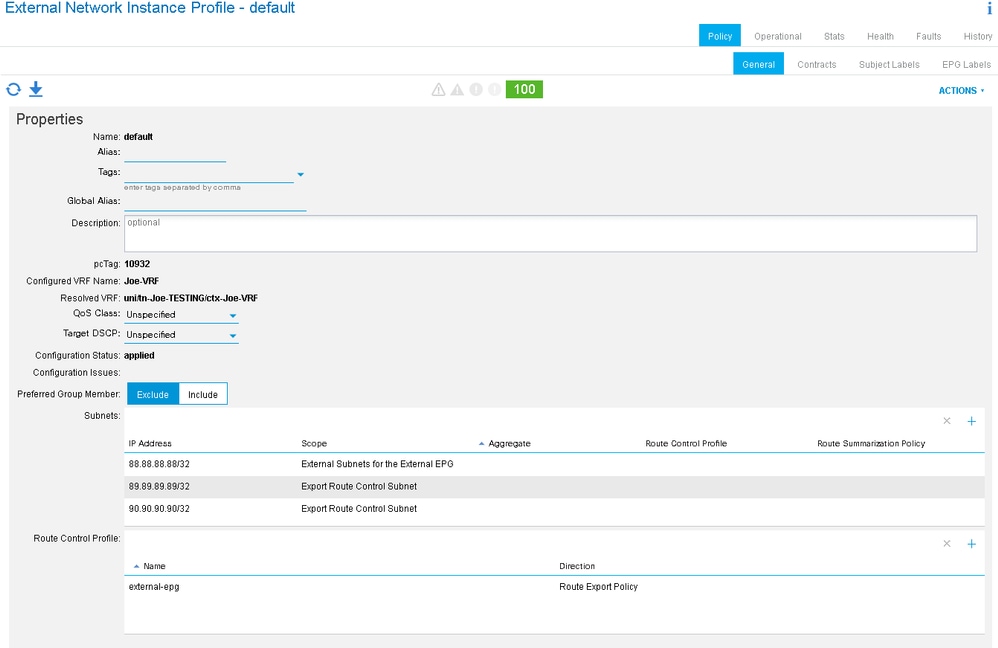This image shows a detailed interface of a web page titled "External Network Instance Profile Default," with a predominantly white header. The layout includes two primary sections identified by blue boxes labeled "Policy" and "General." It's organized with tabs for "Operational Stats," "Faults," "History," "Health," "Contracts," and two additional tabs. Below these tabs, a blue "Actions" label appears, matching the theme of the aforementioned sections.

The main content area is divided into distinct properties listing various details. There is a section with headers "Name," "Default," and "Alias," followed by lines indicating entries for these fields. Tags are indicated by blue lines, and a section for "Global Alias" is similarly marked. A large white box serves as the description area, spanning the width of the page and deemed optional for input.

Further down, another section lists fields such as "Tag Number," "Configured Target," and "Configuration Status," which is marked as "Applied." There is an option for "Preferred Group Master," with choices between "Exclusive" (highlighted in blue) and "Include" (highlighted in white). The page also includes fields for "Subnets" and a "Root Control Profile," each categorized with specific names and descriptors, potentially indicating directional or descriptive information.